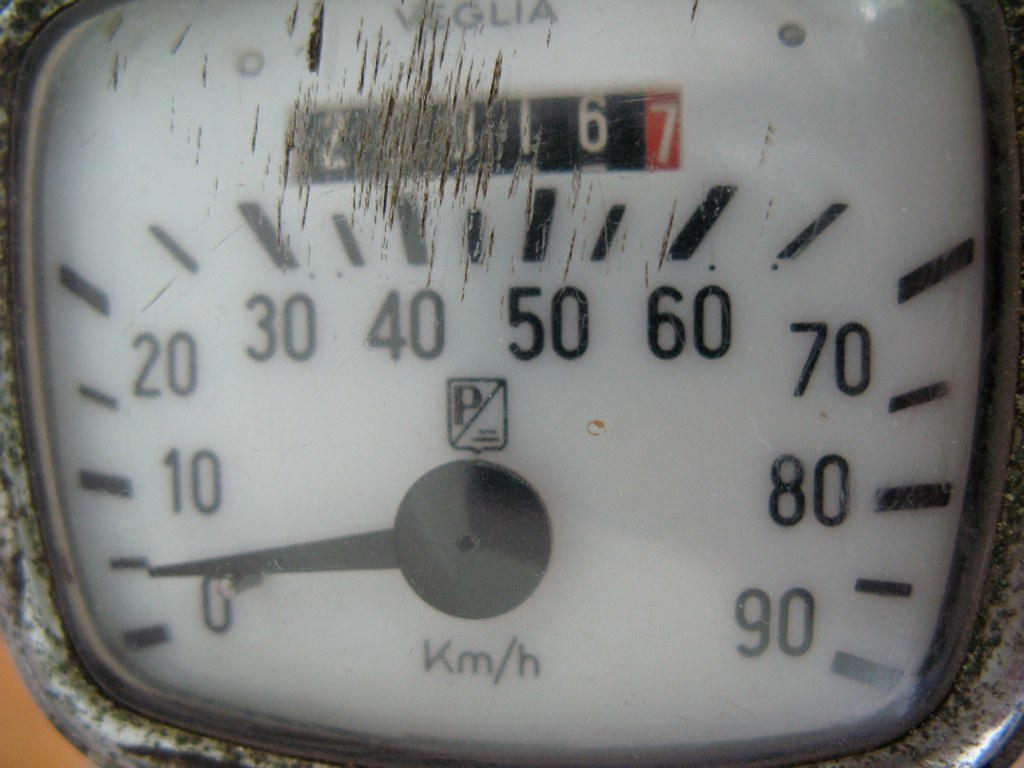A close-up photograph of a vintage speedometer, likely from an older vehicle, reveals its timeworn charm and subtle details. The speedometer is labeled "VEGLIA," though part of the name is scratched and somewhat illegible, hinting at its age. The device features a square design with rounded corners and exhibits significant wear, including deep, dark scratches that obscure some of the readings. 

The mileage display begins with a "2," followed by two sections of unreadable digits, and concludes with "16." The tenths are marked distinctly in red, showing a "7." The background is black with white lettering, typical of older designs, and the measurement is confirmed to be in kilometers per hour (KM/H), as indicated at the bottom.

In the center of the speedometer is a black circle from which an arm or hand extends to point at the current speed, accurately showing approximately 5 kilometers per hour. The speed indicators mark 0, 10, 20, and so on up to 90, with smaller lines indicating increments of 5 units between each main label.

Additionally, a glimpse of the surrounding equipment, possibly part of the headlight holder, is visible, adding context to the vintage vehicle's dashboard setup.